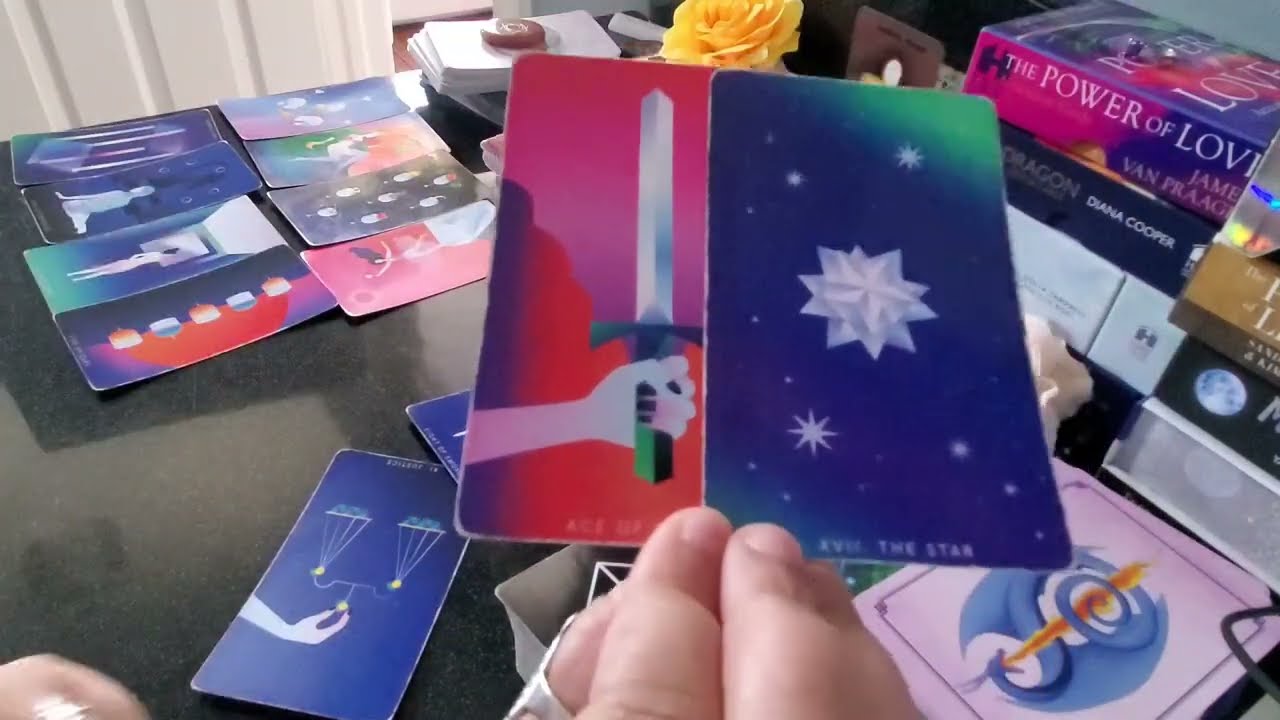The photograph captures a detailed indoor scene centered around a person's hand holding two tall, rectangular cards with curved corners, which appear to resemble tarot cards. The hand is visible from the fingers up and placed at the bottom center of the image. The right card features a blue background adorned with a large, geometric white star in the center surrounded by smaller white stars. The left card, slightly obscured by the right one, displays a graphic design of a cartoon hand gripping a vertical silver sword with a green handle, set against a gradient background from red to pink to purple, with purplish-red clouds and a pink sky.

In the background, there is a shiny black table or countertop covered with several other similar-looking cards spread out, adding to the organized clutter. To the right side of the table, there are towering stacks of books, with visible titles such as "The Power of Love" and "Dragon Something" by Diana Cooper. Additionally, a white door can be seen in the backdrop, along with a messy pile of papers. The overall scene vividly portrays a cluttered yet intriguing setup, likely in a room, hinting at an atmosphere of mystique and exploration.